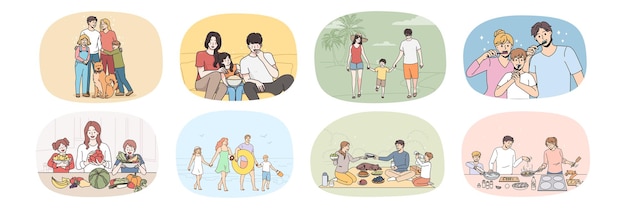This image features eight different cartoon-style scenes of families, each capturing a unique family moment. In the top left corner, a family is hugging each other along with their dog; the man is dressed in a white t-shirt, while the woman with blonde hair wears a red shirt, and they have a boy and a girl. To the right, another family is depicted sitting on a couch watching TV, where the daughter, holding a bowl of popcorn, is nestled between her parents. Adjacent to this, a couple is seen walking on a beach, each holding one hand of their little boy. Another scene shows a family brushing their teeth together, smiling at each other. The image is vibrant with an array of colors including light greens, oranges, yellows, peach, blues, light blues, light pinks, whites, blacks, grays, and red, giving it a lively and warm atmosphere.